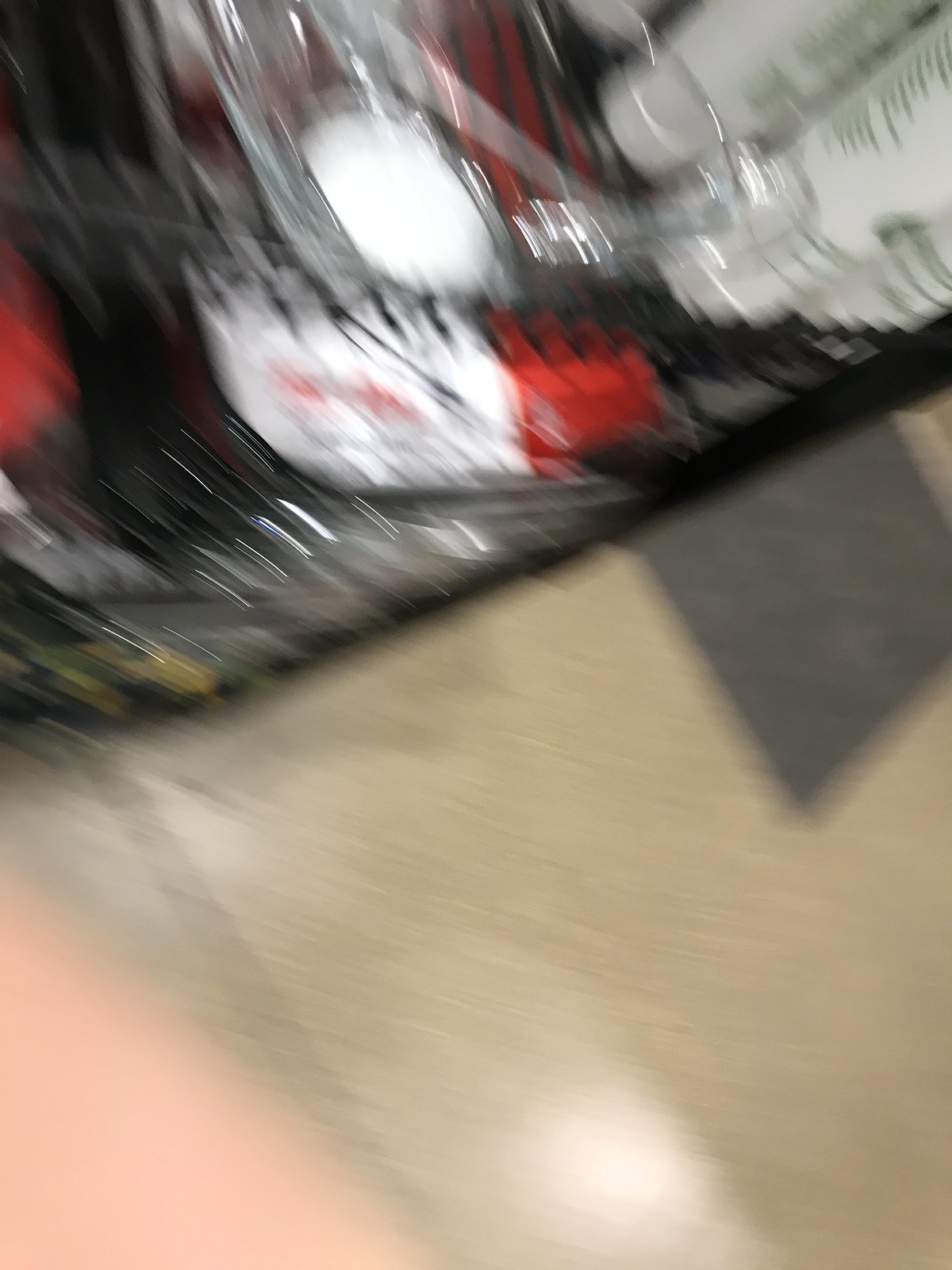A very blurry and low-quality photograph appears to capture the bottom edge of a black metal shelf with thin, open bars. The camera angle is tilted, and the floor beneath the shelf is predominantly white tile, featuring a distinctive large gray tile. The shot focuses on the bottom three shelves, which hold a variety of indistinguishable items. Among these, black paper plates are clearly visible. Other items on the shelves include vague assortments of paper and plastic goods, some of which are clear bottles and red objects. A white container with red writing, rendered illegible by the blur, is also present. The overall impression is one of motion, as if the camera was accidentally moved or dropped while the photo was taken, resulting in the significant lack of clarity.